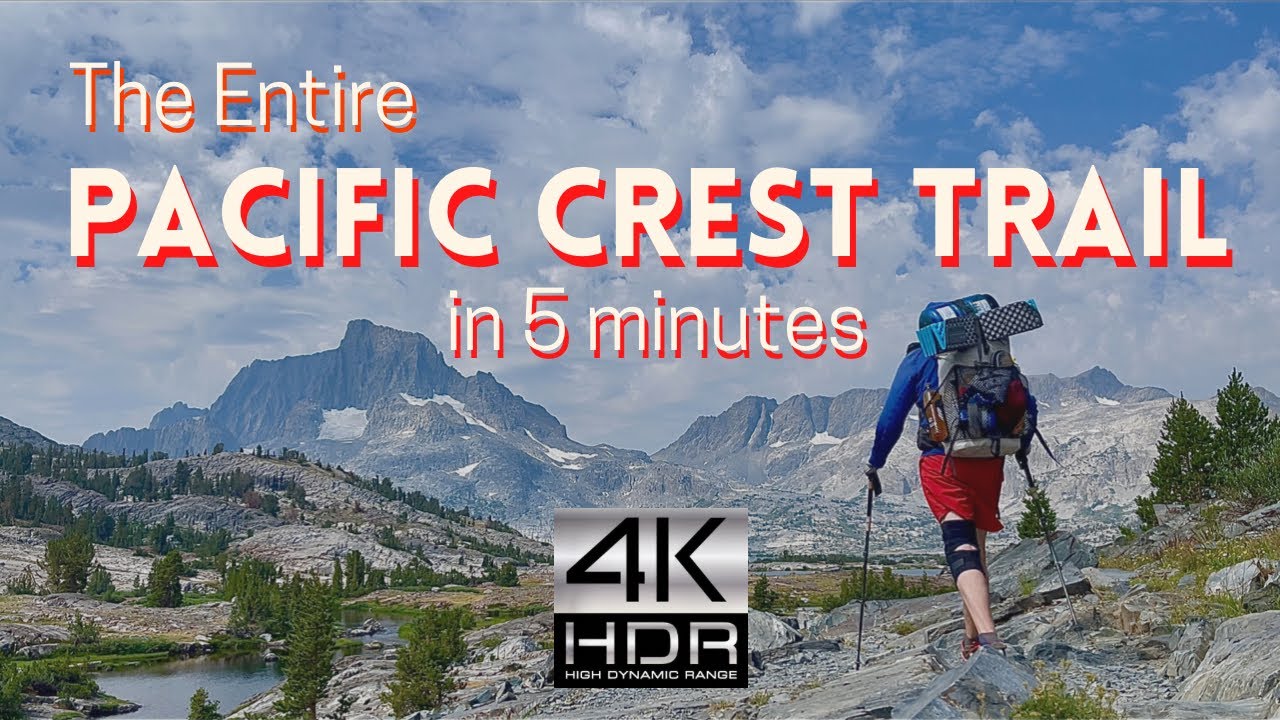The image resembles a YouTube video thumbnail and prominently features the text "The Entire Pacific Crest Trail in 5 Minutes" in white font outlined in red. Below this, there's a logo indicating "4K HDR," which promises high dynamic range resolution for the video. In the foreground to the right, a Caucasian hiker is visible, geared up with a large backpack, a blue windbreaker, red shorts, and a black knee brace on his left knee. He is equipped with two metal hiking poles. The hiker navigates a rugged, rocky terrain with jagged gray rocks and patches of green grass and weeds. The background showcases tall, jagged mountain ranges with snowy peaks, thick pine trees, and a winding river on the left side of the image, all under a partly cloudy blue sky.